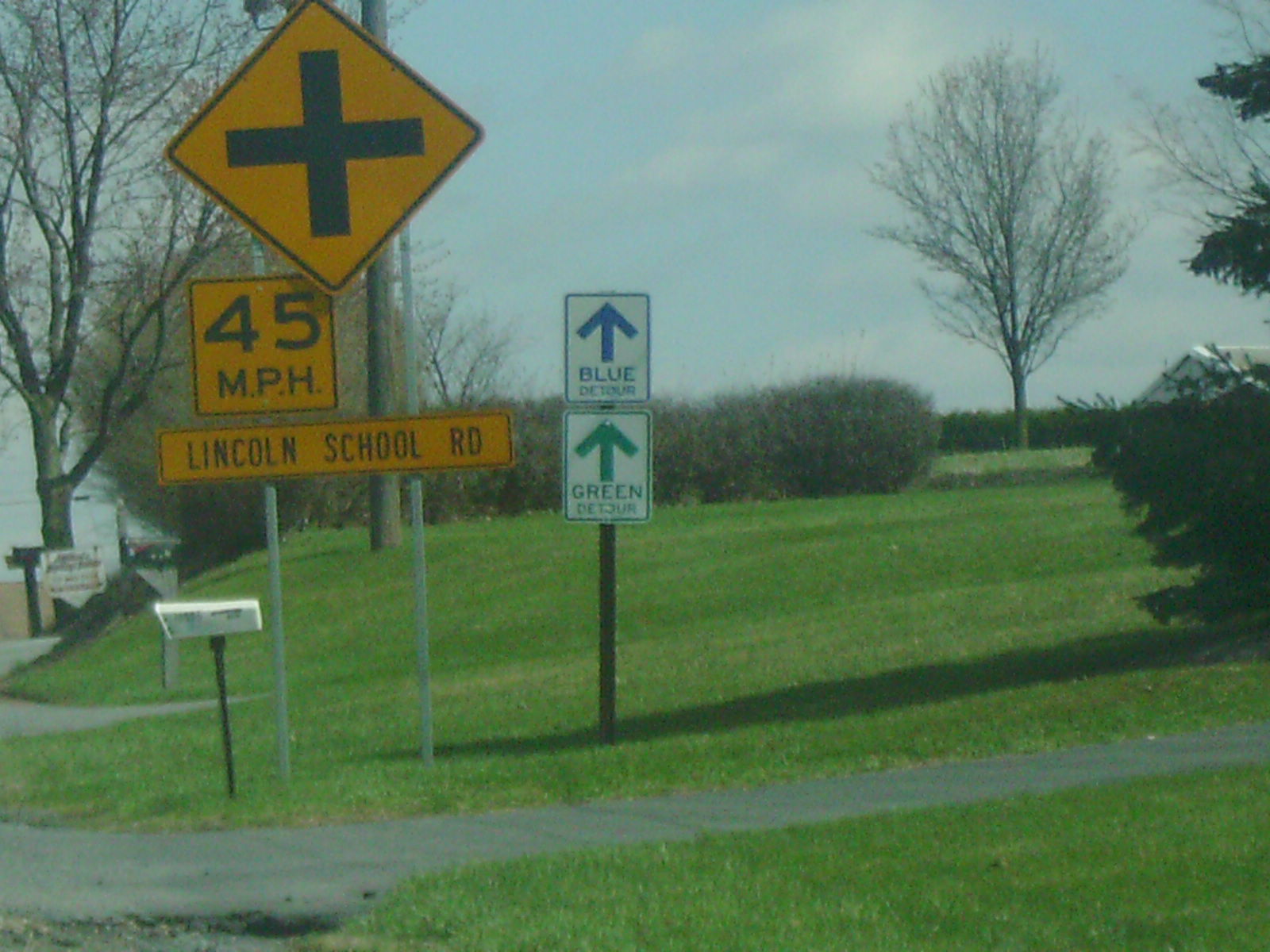This outdoor photograph captures a roadside scene featuring various signage against a backdrop of sloping green grass, shrubbery, and leafless trees, suggesting a transition between seasons, either late autumn or early spring. The focal point is a prominent yellow and black sign indicating an upcoming crossing at Lincoln School Road, with a speed limit of 45 miles per hour. Flanking this main sign are two detour signs: a blue arrow and a green arrow, hinting at alternate routes ahead. Adjacent to the signage is a white mailbox, adding a touch of rural character to the scene. The overall composition effectively conveys a navigational crossroads surrounded by nature.